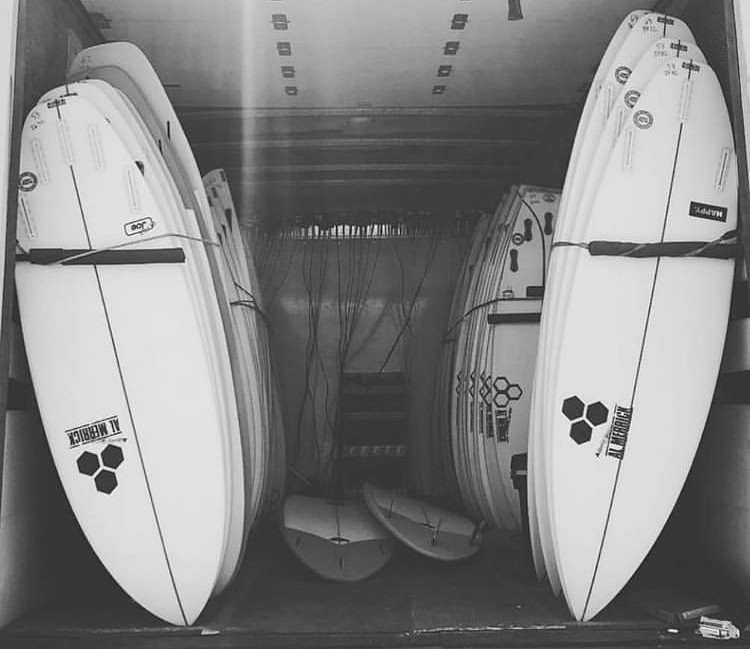The black-and-white photograph captures a large number of surfboards stacked upright on their pointy ends, varying in size, and carefully bound together with ropes. They are positioned in the back of what appears to be a trailer or garage with an open sliding door above them. The trailer, resembling a U-Haul, has a strap hanging from the door, which has been slid up to reveal the interior. From the back of the trailer, you can see a window at the front that lets in some light, along with some wires dangling from the ceiling. The surfboards, while roped together, appear precariously stacked but may have padded sheets to prevent damage. The overall image exudes a vintage feel with its black, white, and gray tones, and there is a sense of organized chaos in the confined space.